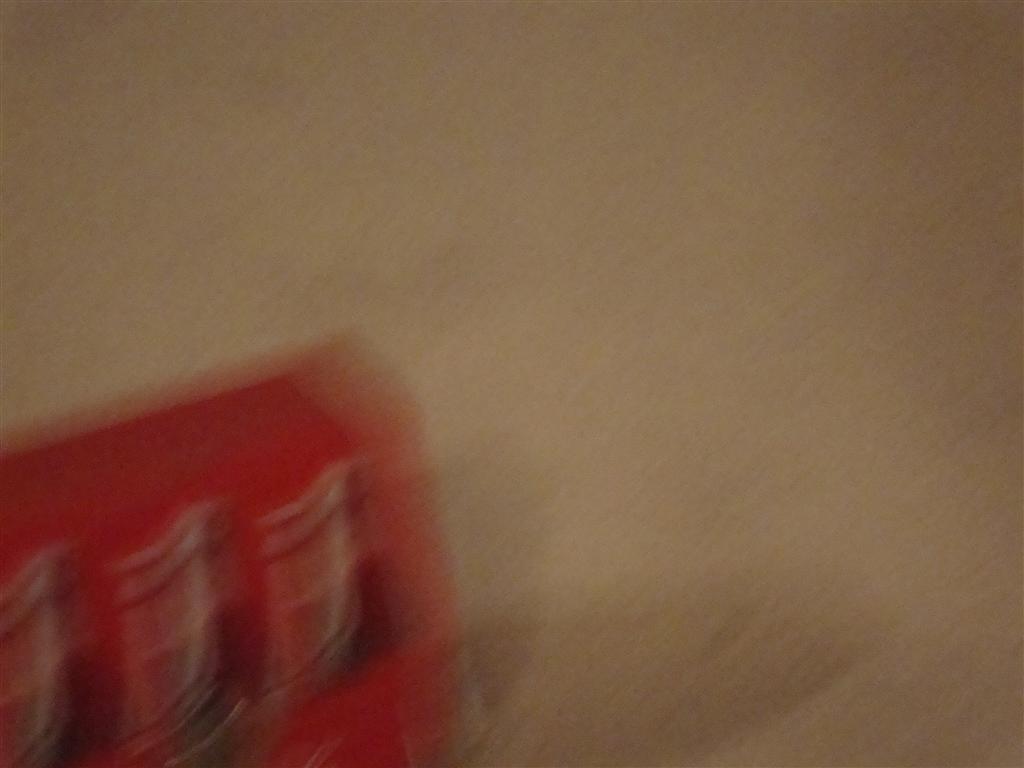The image features a light brown background with a red and white checkered square positioned in the lower left corner. The square is divided into three distinct sections. The brown surface displays subtle grains and variations in color, including white specks and darker borders, giving it a textured and slightly shadowy appearance. The red square casts gentle shadows onto the brown background, enhancing the depth and contrast within the composition.